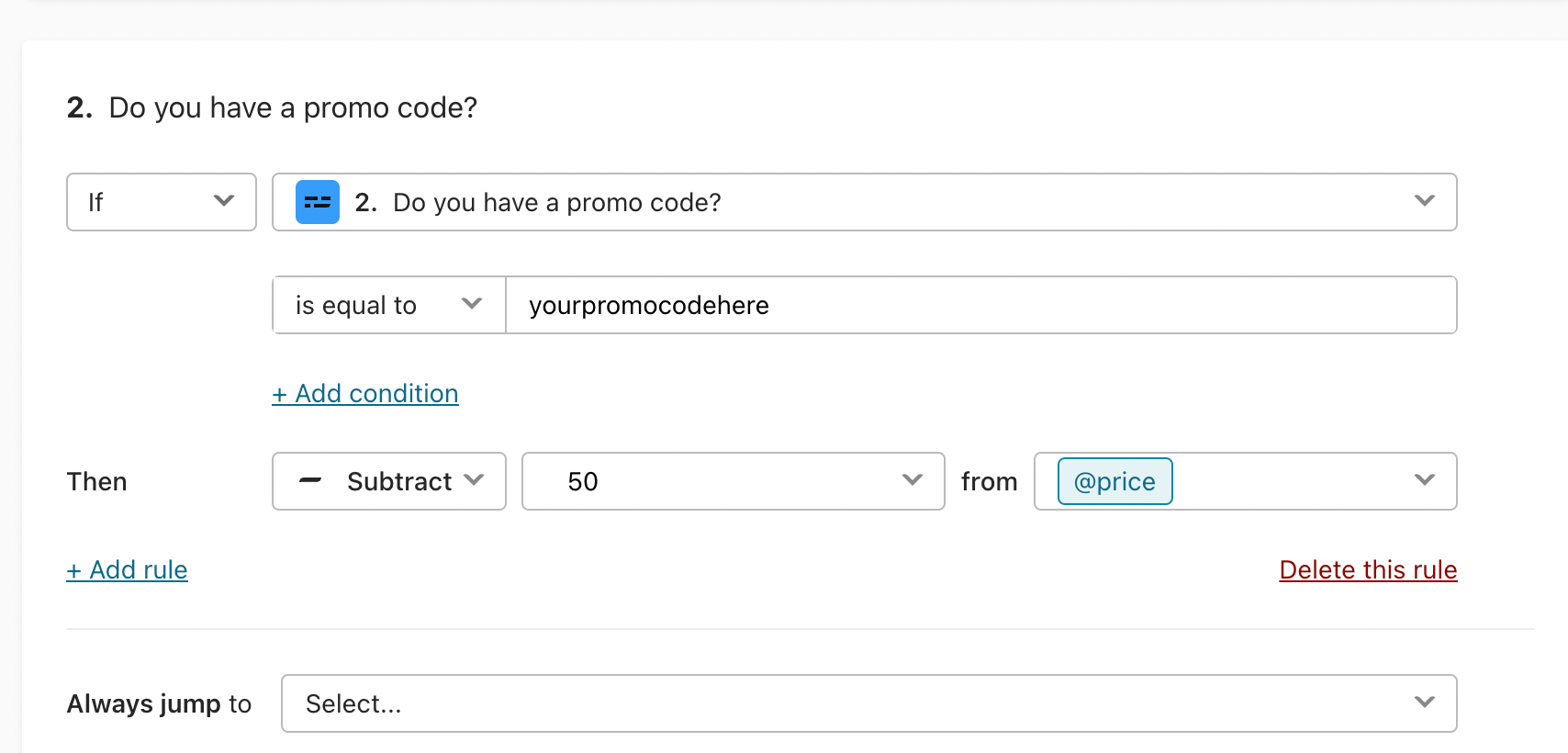**Caption:**

This image depicts the settings page of an e-commerce platform for configuring a promotional code. The interface features a simple design with a gray background and white text areas, outlined by thin gray lines. At the very top, a text block is partially visible, with its content cut off. Below it, labeled as "Number 2," the question "Do you have a promo code?" appears within a dropdown box. Adjacent to this dropdown, another dropdown is set to "if," followed by yet another dropdown box asking "Do you have a promo code?" with a question mark.

Beneath this, there's a dropdown stating "is equal to," accompanied by a text field which contains the placeholder text "yourPromoCodeHere." A link nearby prompts users to "add a condition." Further down, a logical condition is set up with dropdown boxes: one set to "subtract," another to "50," and a following one indicating "from." This is visually represented by a tagged, rounded rectangle box labeled "at price."

At the bottom of the interface, users have options to "add a rule" and "delete this rule," along with additional text at the very bottom stating "Always jump to," paired with a dropdown box that is currently set to "select."